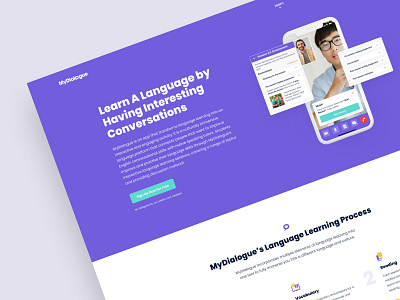The image appears to be a low-quality, off-center screenshot, likely taken from a website, featuring a piece of paper or digital flyer on a gray background. The top portion of the flyer is a blue or purple shade with text in white font. Prominently displayed in large capital letters, it reads, "Learn a language by having interesting conversations." The top left corner of the flyer has blurry, small text that seems to say "my dialogues," but it is difficult to decipher. The image also includes a depiction of a cell phone screen showing two individuals engaged in what appears to be a FaceTime video call, possibly for language learning purposes. The bottom of the flyer has additional information detailing the "my dialogues language learning process," but this text is too small to read clearly. The overall layout suggests this could be promotional material for a language learning application focused on conversational practice.